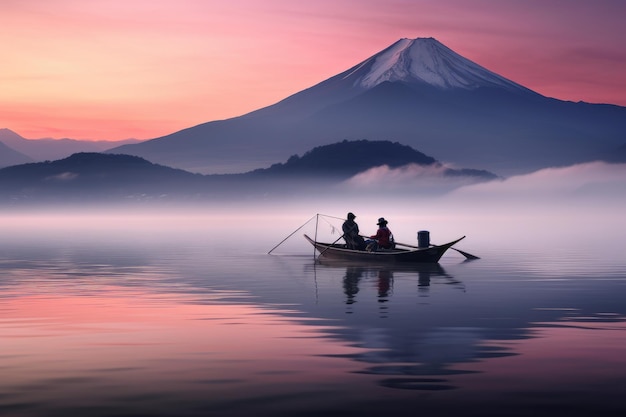This detailed painting, which closely resembles a realistic photograph, captures a serene twilight scene. At the bottom of the image, a somewhat wavy water body reflects the painting's colors. In the water, a small boat carrying two people is visible; they appear as silhouettes due to the dim, failing light. The figures are rowing the boat, possibly equipped with rods or oars, hinting that they might be fishermen. The backdrop features a mist-covered mountainous landscape, with hills in the foreground and a prominent volcanic mountain rising in the distance, its peak capped with snow. The sky is awash with hues of purple, pink, orange, and yellow, casting a reddish glow that is mirrored on the water's surface, enhancing the ethereal quality of the scene.